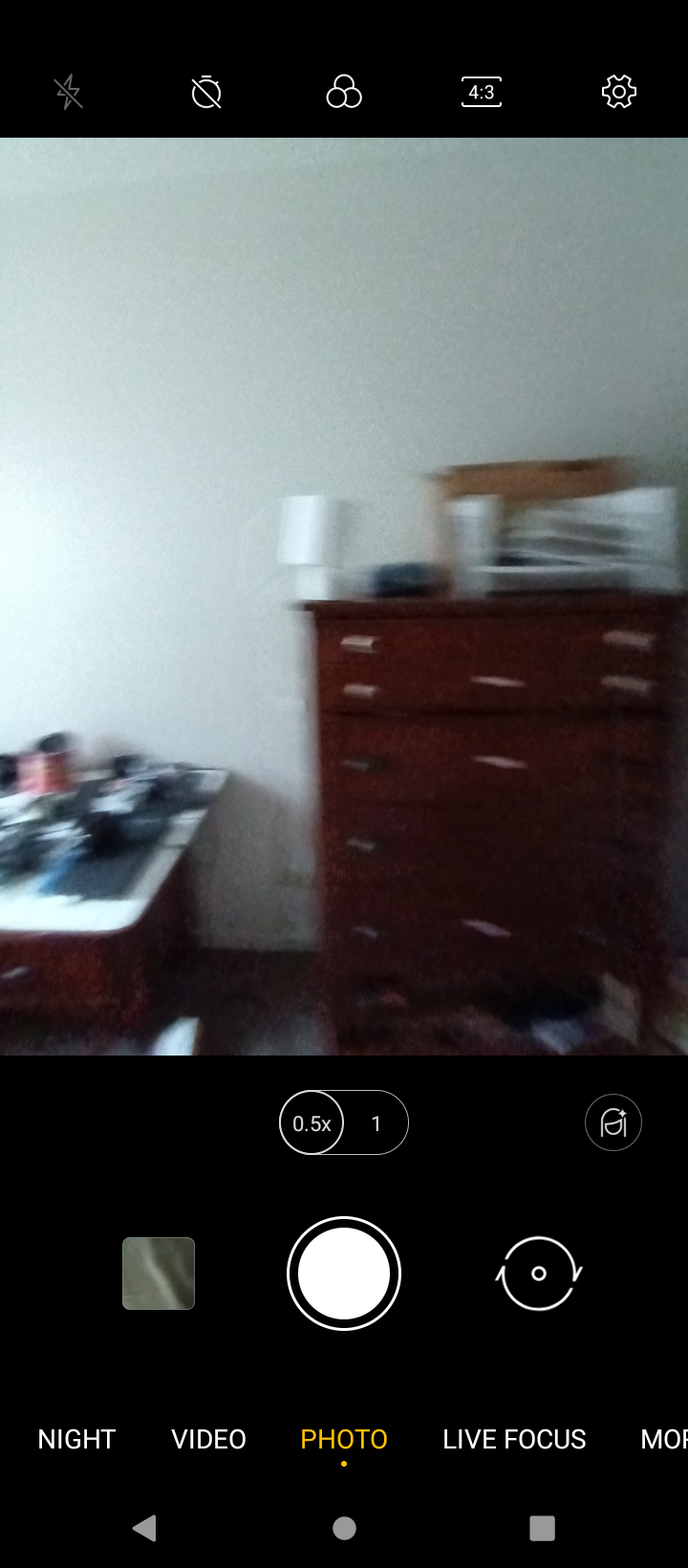This image showcases a smartphone screen with a black status bar at the top, featuring a series of icons arranged from left to right. The first icon is a flash symbol with a gray diagonal line through it, indicating the flash is turned off. Next to it is a white circle with a diagonal line, commonly representing a generic prohibition or "do not" sign. Following that, there is an icon showing three circles arranged in a triangular pattern, with two at the bottom and one at the top. Moving further to the right, there is a text segment displaying "4:43," suggesting the current time. To its right is a settings icon shaped like a white gear. Below this status bar, the majority of the screen displays an image. The image seems to feature part of a room, visible is a white wall and a drawer situated on the right side of the frame.